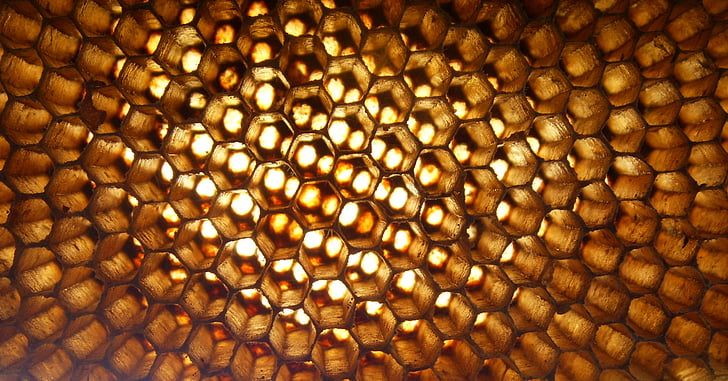The image portrays a horizontal, rectangular close-up of numerous gold-colored, round-shaped items meticulously arranged in a geometric pattern, completely filling the frame. The lighting emphasizes a gradient effect, with the central region radiating a bright, golden-yellow hue, while the peripheral areas appear in darker shades of brown and tan. The repetitive alignment of these interconnected shapes resembles the inside of a honeycomb, contributing to a visually intriguing and symmetrical pattern. The overall artistic composition, complemented by the light's central highlights creating almost rays of light, remains open to interpretation, evoking thoughts of both a scientific object and a piece of abstract art.